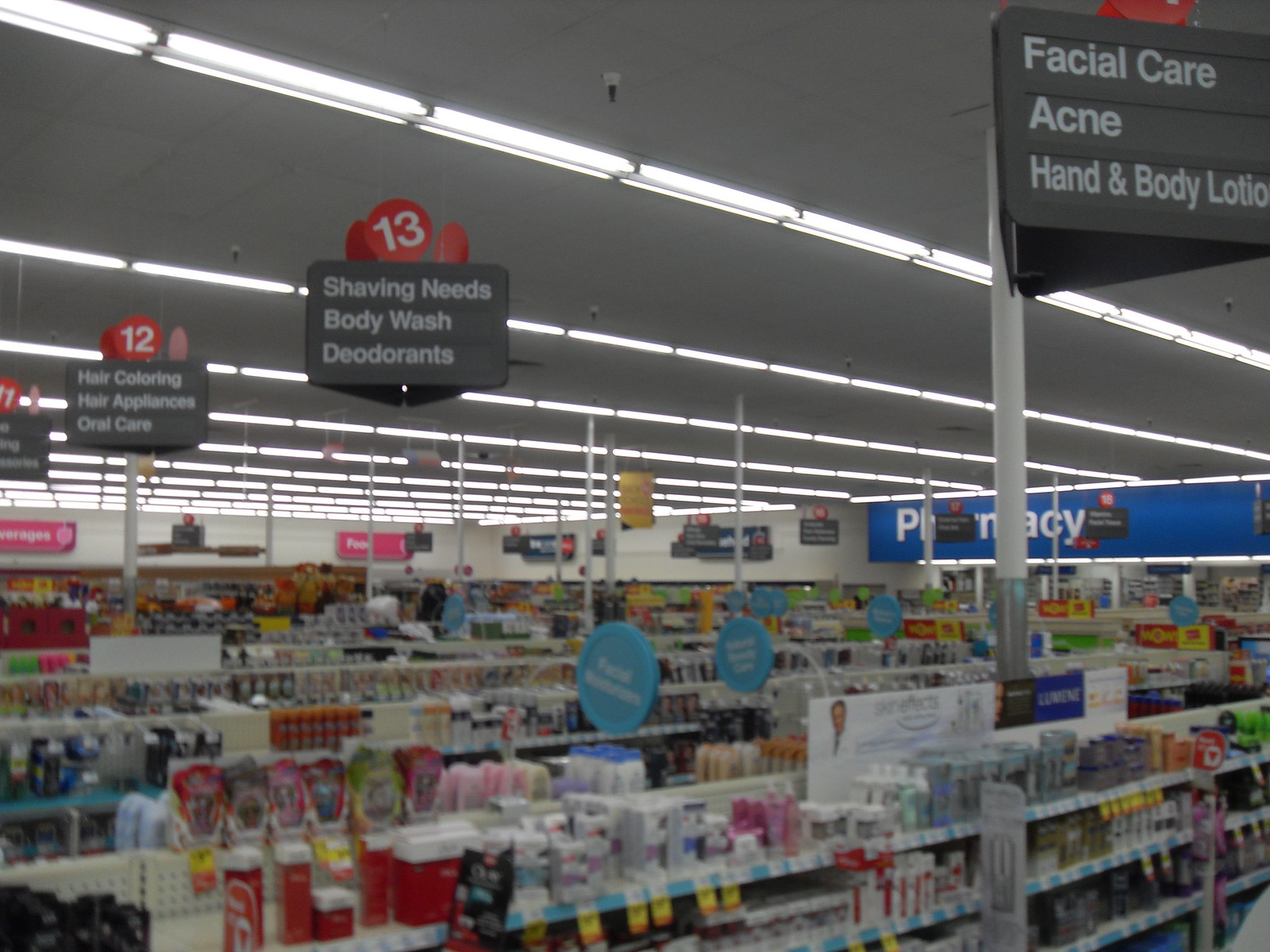The image depicts the interior of a retail store, most likely a CVS pharmacy, as viewed from an elevated angle. A series of short, neatly arranged shelves extend from the lower left to the center right of the frame, filled with various personal care products. Above these shelves are gray aisle signs with white text, indicating the categories of items available, such as Hair Coloring, Hair Appliances, Oral Care, Shaving Needs, Body Wash, Deodorants, Facial Care, Acne, and Hand and Body Lotion. Aisle number markers, featuring red circles with numbers like 12 and 13, appear on top of these signs. In the back right corner, a large blue banner with white text, partially obscured by signs and poles, indicates the Pharmacy section. Fluorescent lights are arranged in rows across the ceiling, providing bright illumination throughout the store.